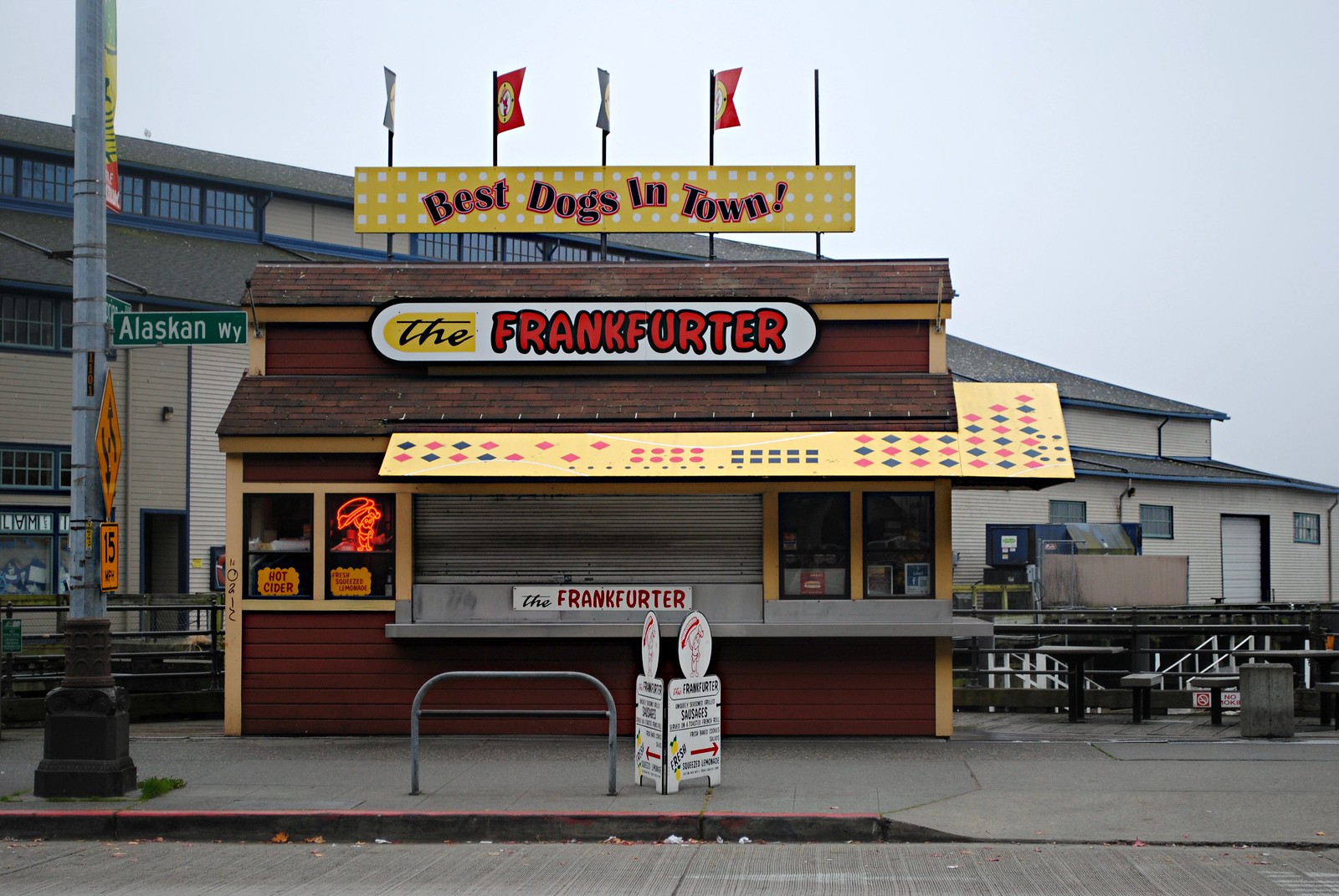In the daytime photograph of a small town, we see a quaint hot dog stand nestled on a sidewalk. The photograph is wider than it is tall, measuring approximately five inches in height and six inches in width. In the foreground, a gray street with fine, horizontally raised grating meets a curb marked by a red stripe. The curb features an accessible ramp on the right side, designed for wheelchair use.

On the left side of the image, a tall metal post supports several street signs. Among them, an orange sign displays the number 15, a diamond-shaped sign shows some arrows, and a green rectangular sign with white lettering reads "Alaskan W.Y." 

Dominating the scene, the hot dog stand has a distinctive, rustic charm, evoking a barn-like appearance with its yellow, red, and black coloration. Atop its slanted brown roof wave four or five small flags. Beneath these flags, a prominent rectangular sign boasts a yellow background with white squares and declares in black print outlined in red, "Best Dogs in Town."

Further down on the stand, another sign features the word "The" in black cursive on a yellow background, followed by "Frankfurter" in bold red letters with black outlines. This sign is affixed beneath a light tan or yellow awning adorned with black and red geometric patterns including squares, circles, and diamonds. 

The hot dog stand appears to be closed, as indicated by a metal roll-down door covering the serving area, which also bears the name "The Frankfurter." Adjacent to the stand, concrete seating areas are visible, offering potential seating for customers. In the background, a large tan building with dark windows looms, contrasting against the gray-blue sky above.